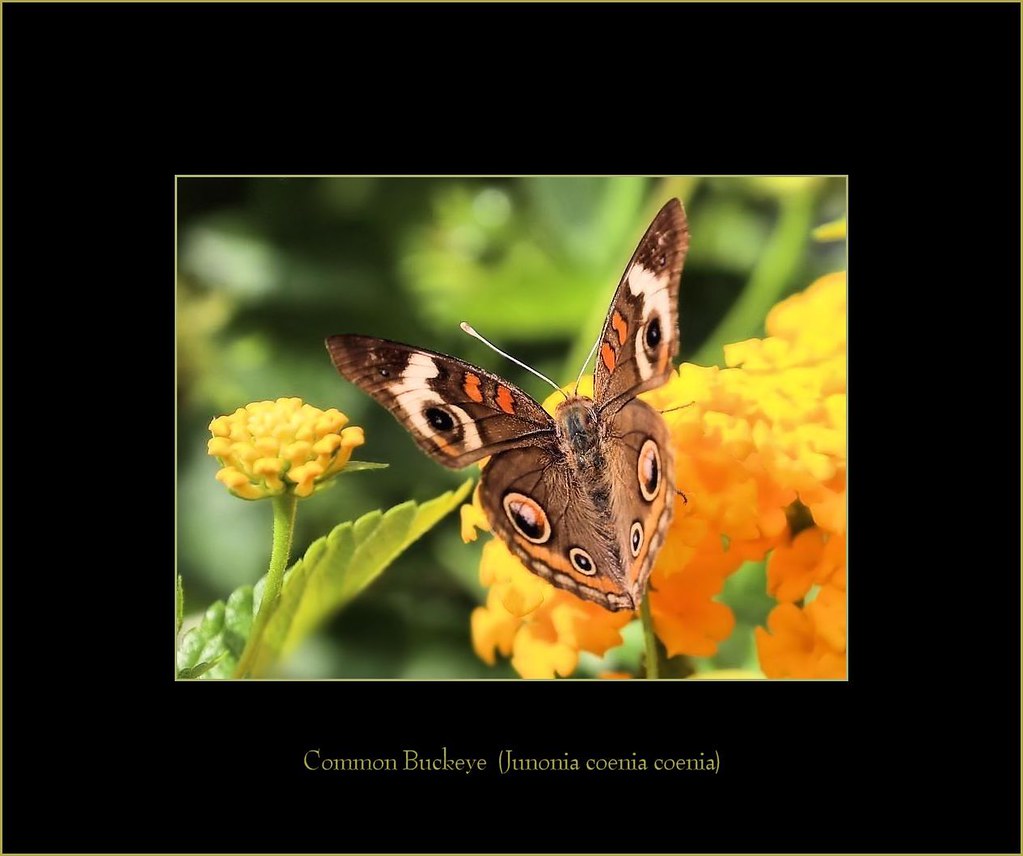The image is a striking, colorful photograph of a Common Buckeye butterfly (Junonia coenia) resting on small, bright yellow flowers that resemble cauliflower. The butterfly is predominantly brownish-orange, with intricate wing patterns that include three eye-like spots on each wing, totaling six eyes. These eyes are not only colorful but resemble cat eyes, adding to the butterfly's defense mechanism. The butterfly is framed by lush green leaves and stems around the flowers. The photo, which is bordered in yellowish-gold and set within a black frame, has text at the bottom that reads "Common Buckeye" in yellow font, with the scientific name "Junonia coenia" in parentheses. The background is a blur of green, suggesting a garden or natural setting rich with plant life.